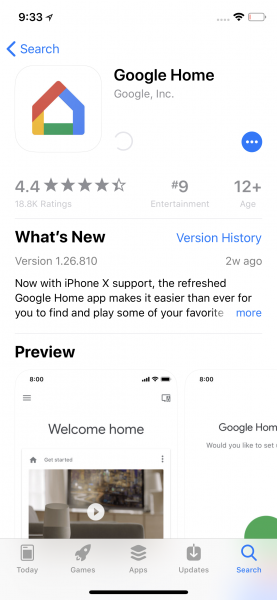A screenshot from a smartphone displays the Google Home website. At the top-left corner, the screenshot shows the time "9:33". On the right side, there are icons for Wi-Fi connectivity and battery status, with the battery icon indicating it is nearly empty. Below this, there's a search bar featuring an arrow pointing to the left and the word "Search" in blue.

Centrally positioned in black letters, it reads "Google Home, Google Incorporated," accompanied by a square logo featuring a red, blue, green, and yellow house-shaped image. The Google Home page holds a 4.4-star rating from 18.8K reviews, is ranked number 9 in the Entertainment category, and is recommended for ages 12 and up.

Under "What's New" and "Version History," it states the app's version as 1.26.810, updated two weeks ago. The partial description reads, "Now with iPhone X support, the refreshed Google Home app makes it easier than ever for you to find and play some of your favorite...", with the sentence abruptly ending.

Displayed towards the bottom of the page are previews of the app and icons for "Today," "Calendar," "Games," "Apps," "Updates," and "Search."